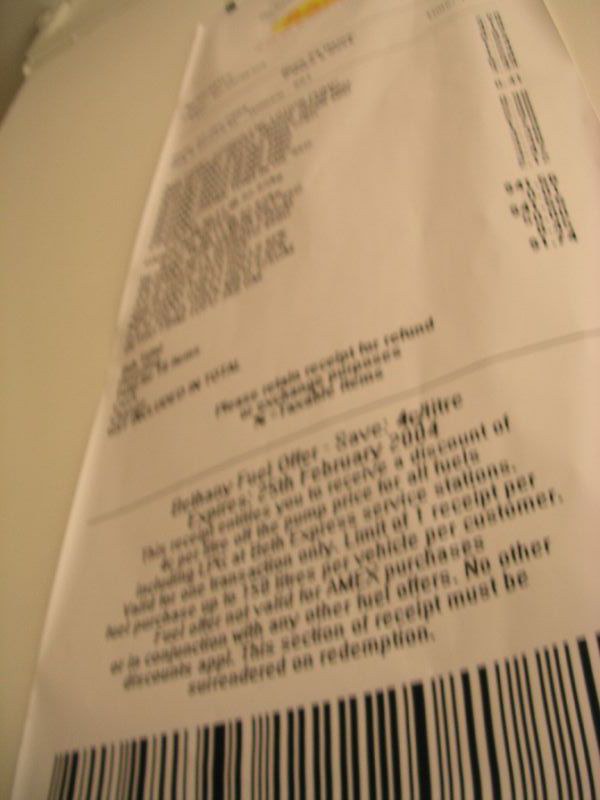This image depicts a blurry and distorted photograph of a long, rectangular paper receipt, typed in black ink. The receipt lists multiple purchased items, forming a vertical stack of largely illegible numbers and descriptions. The fonts toward the bottom appear larger, making certain details somewhat more discernible, such as a total amount and promotional text mentioning an expired offer for 4 cents per litre on fuel. An especially visible section towards the end of the receipt states "expires on the 25th of February 2004." There is a large barcode at the bottom, adding to the indication that this is indeed a receipt. Additionally, a small section near the top is tinged yellow, possibly due to highlighting or a yellow print. The receipt rests on a white surface, suggesting a white table beneath it, and the photo was taken in a dimly lit room. Despite the poor focus and clarity, the black lettering on a white background is consistent throughout the image.